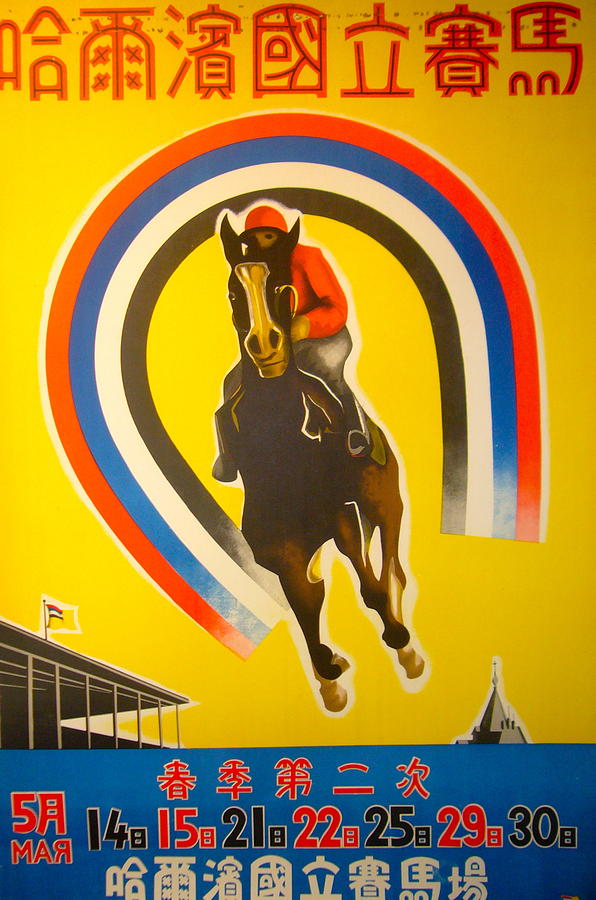The image depicts a vibrant, printed poster featuring a yellow background. Dominating the top half are large, bold Chinese characters in red. A prominent upside-down horseshoe frames the illustration with striking stripes in black, white, blue, and red. At the center, a brown horse with golden markings on its snout gallops forward, ridden by a jockey dressed in a red helmet, red jacket, white pants, and black boots. The jockey's attire, combined with the dynamic positioning of both horse and rider, conveys a sense of motion and vigor. The bottom of the poster features a blue highlighted bar containing additional Chinese text and a series of numbers, notably including dates such as March 5, and numerals like 14, 15, 21, 22, 25, 29, and 30, written in red, black, and white. The entire composition is accented by a diverse palette and intricate details, merging cultural elements with the high energy of horse racing.